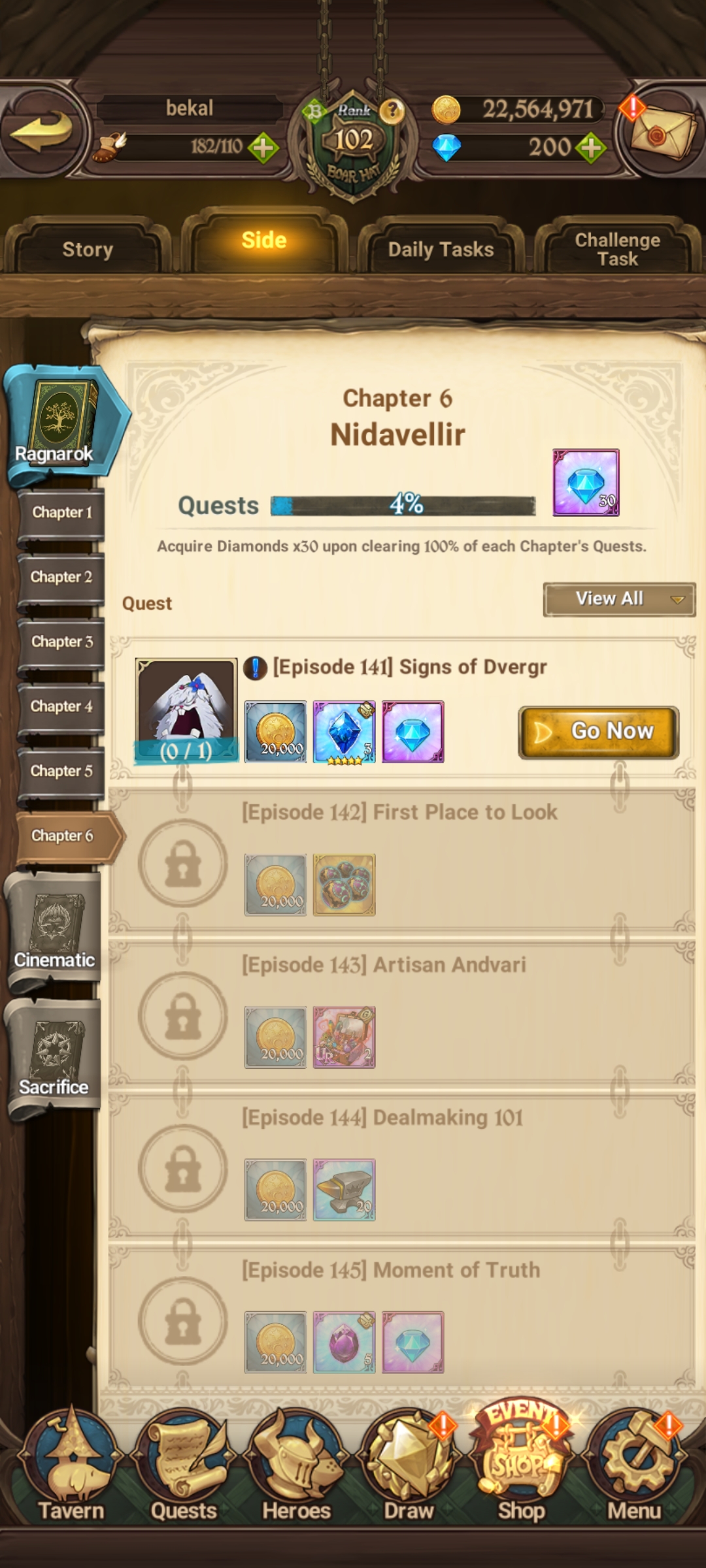This image is a detailed screenshot of a medieval-themed gaming app displayed on a phone. At the top quarter of the screen, there is a light brown area with some writing that appears slightly out of focus, possibly displaying the user's name. Below this section, there are various indicators including a diamond icon with the figure "102," a coin counter showing "22,564,971," and a blue diamond symbol marked "200." On the right side, there is an icon resembling a knapsack.

The center portion of the screen features navigation tabs for different game modes and tasks. From left to right, these tabs include "Story," "Side" (currently highlighted), "Daily Tasks," and "Challenge Tasks." Below this, there are various outfits or in-game unlocks displayed.

The bottom of the screen is lined with different functional tabs including "Tavern," "Quests," "Heroes," "Draw," "Shop," and "Menu." The game display indicates it is on Chapter 6 titled "Native Valaire," with quest progress marked at 4%. The left side of the screen shows all available chapters, giving the interface a cartoonish medieval appearance.

Overall, the image captures a detailed and immersive interface of a medieval-themed mobile game.